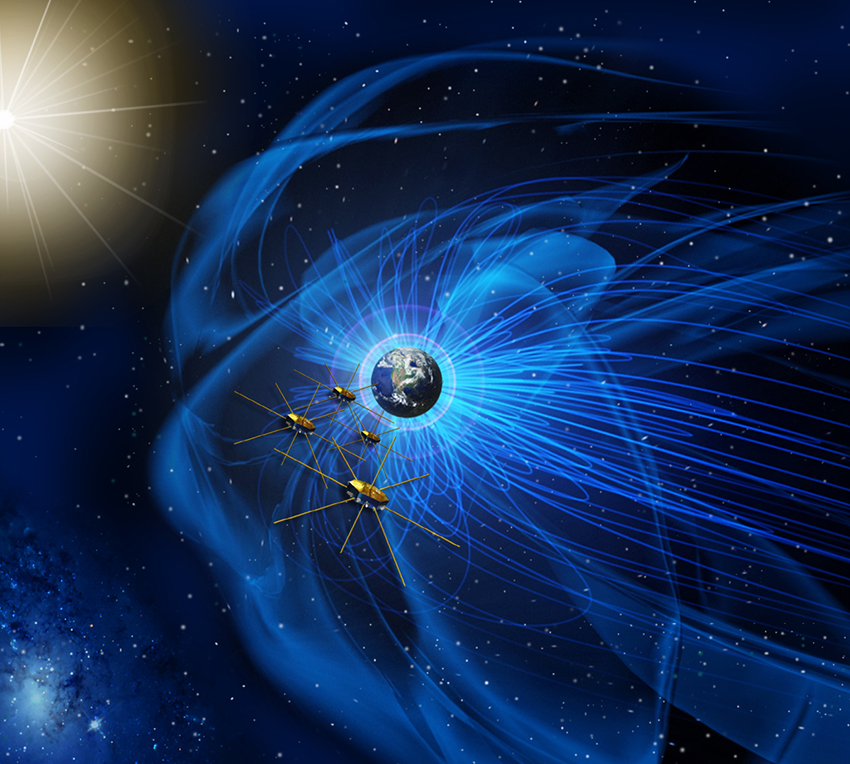This is a highly detailed, digitally-created painting depicting an outer space scene. The dark, black, and blue expanse of space is scattered with small, gold stars. Dominating the center of the image is the Earth, portrayed with vivid detail: it's blue with swirling white clouds and features orange and green landmasses. Surrounding Earth are swirling ribbons and vortices of blue gas. On the top left, a bright, shining sun illuminates the scene. In the foreground, there are four gold-colored structures resembling satellites, each with circular disks and antennae, seemingly directed towards Earth. The bottom left corner captures part of a galaxy with a striking blue vortex-like appearance, while the rest of the background continues to showcase the star-speckled, black cosmic void. The overall image lacks textual elements, focusing purely on its visual storytelling.